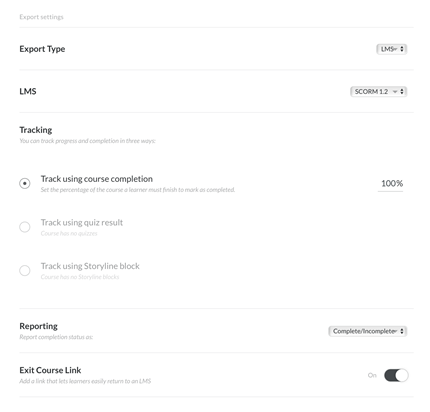This image is a detailed screenshot of an LMS export settings chart. At the top of the chart is a blank line. Below this, on the left side, is the heading "Export Settings" in bold. The next row is labeled "LMS," followed by "Tracking." Under the "Tracking" row, there is a subtext in smaller gray font that reads, "You can track progress and completion in three ways." Three options are listed, with the first one selected: "Track using course completion." The other two options, which are not selected, are "Track using quiz results" and "Track using storyline block." 

The subsequent row is labeled "Reporting," and the final row is titled "Exit Course Link." All row titles are in bold black letters. On the right side of the chart are various interactive elements like scroll bars and drop-down menus: 

- For the "LMS" row, there is a drop-down menu on the far right with "SCORM 1.2" selected.
- For "Export Type," a similar drop-down menu shows "LMS" selected.
- For "Tracking using course completion," it shows 100% completion.
- For "Reporting," the drop-down menu displays "Complete/Incomplete" as the selected option.
- The "Exit Course Link" is toggled on. 

There is a considerable amount of white space between the left-aligned text and the values on the right.